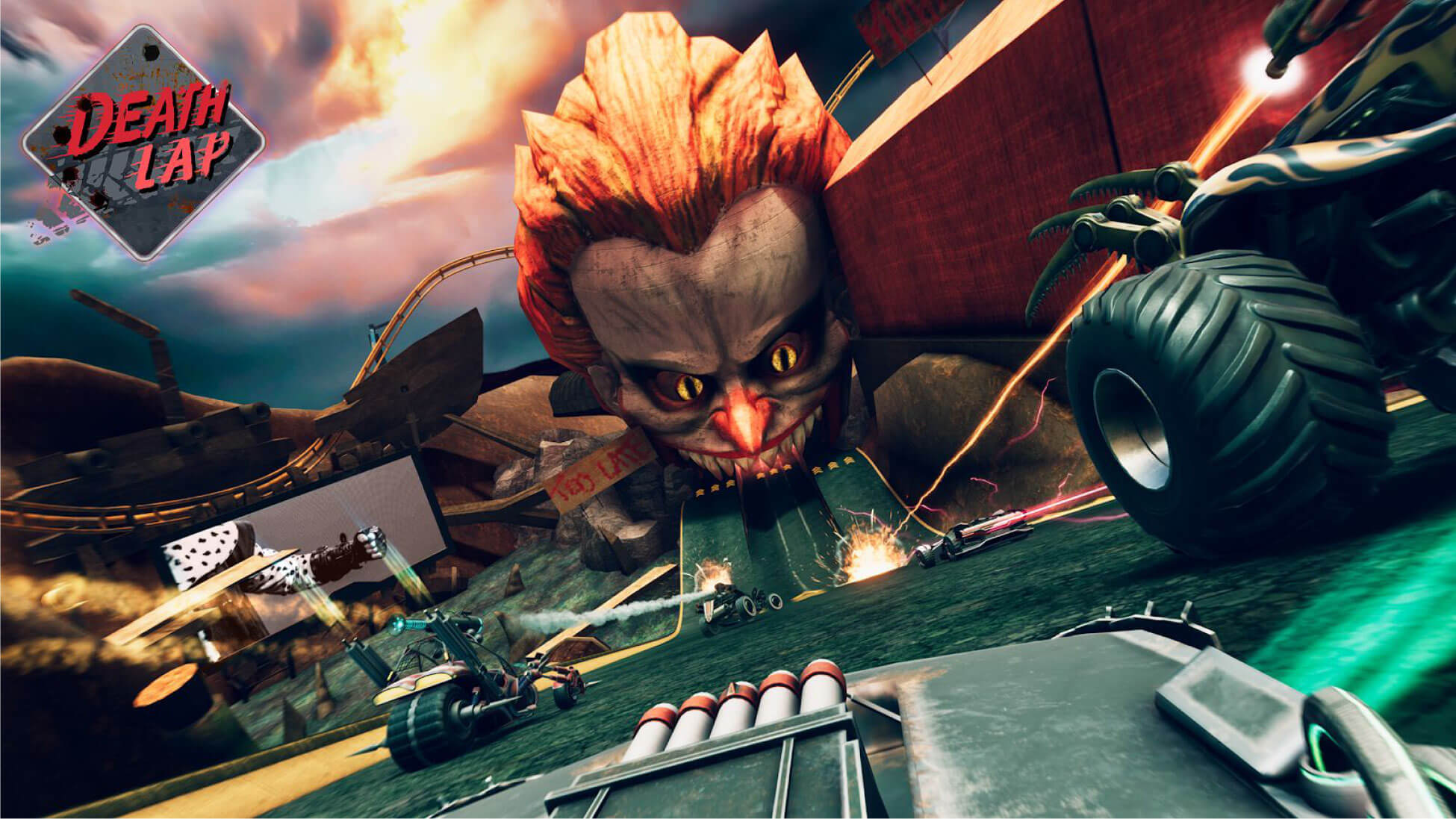The image captures an intense moment from a video game depicting a chaotic car battle. The scene is set against a grayish, cloudy sky tinged with orange and pink tones. In the upper left corner, a diamond-shaped background highlights the red text "DEATH LAP." Dominating the horizon is an ominous, towering clown face with striking orange hair, a sharp orange nose, yellow cat-like eyes, and a menacing grin with white teeth and red lips.

In the foreground, five vehicles are converging towards the clown face. The vehicles are varied, including cars and motorcycle-like hybrids, armed with distinctive features such as large wheels, claw-like appendages, and lasers. The vehicle closest to the camera, which itself is mounted on another car, sports a prominent laser emitting a red beam. The entire scene evokes a high-stakes race or battle, accentuated by a racetrack that seems to emerge from the clown's gaping mouth, adding to the eerie, adrenaline-pumping atmosphere.